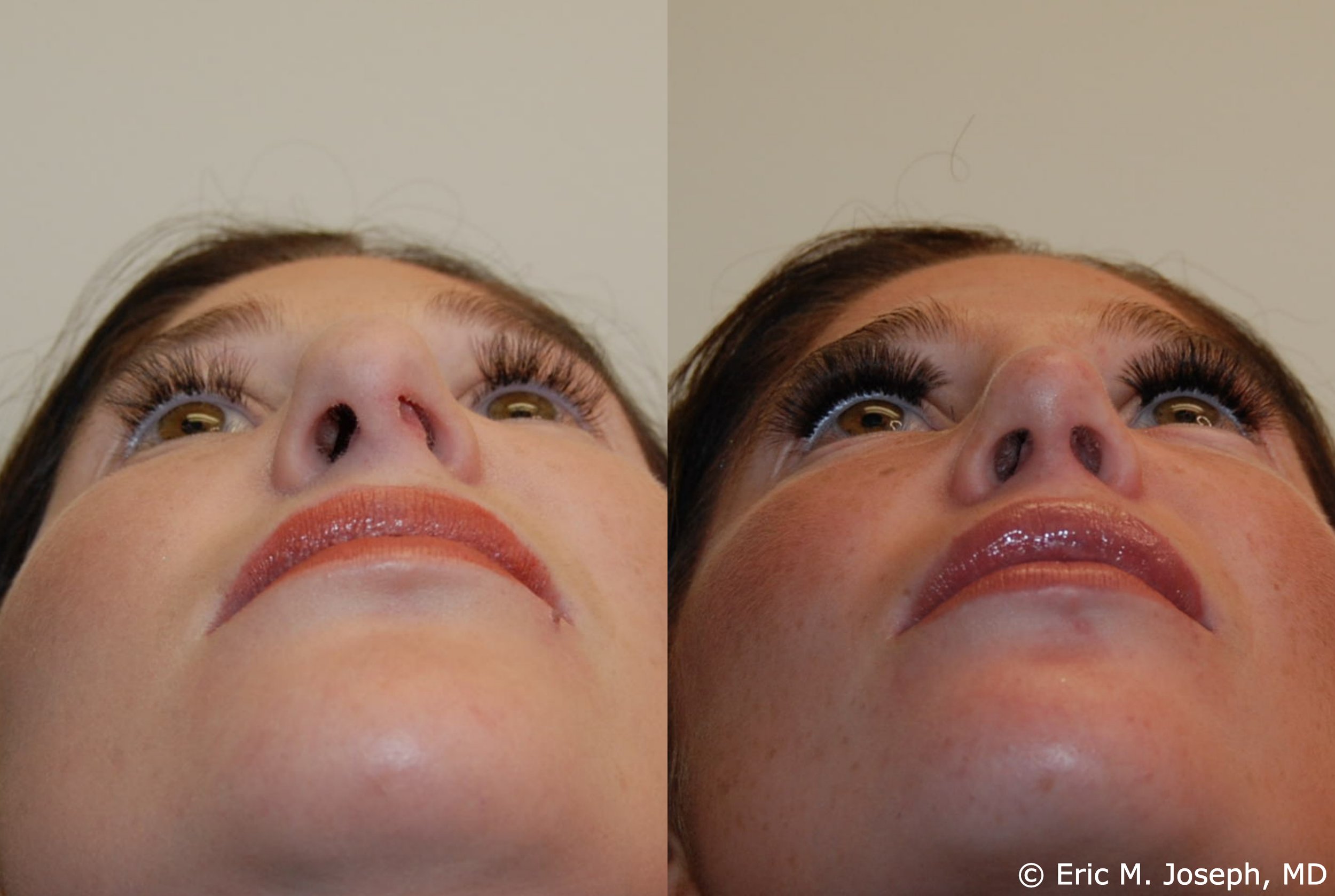The image is a side-by-side comparison of a woman's face, taken from a lower angle, looking upward towards the ceiling. In the left-hand photo, her skin appears lighter and fresher, but there is noticeable obstruction in her nasal airway, possibly due to excess skin. Additionally, some of her hair strands are separated, and her eyebrows are thinner. Her eyelashes and mascara are less prominent as well, and she has a lighter application of lipstick. 

In the right-hand photo, her nose appears to have healed and is more open, indicating a possible medical intervention by Eric M. Joseph, MD, whose credit is noted in the bottom right corner. This photo has a warmer tone, with red blotches visible on her cheeks, chin, and under her lips, suggesting a recent cosmetic procedure or skin irritation. Her eyebrows are fuller, and she is wearing darker, fuller lipstick along with more pronounced eyelashes or mascara.

Overall, the comparison highlights the changes in her nasal structure and facial aesthetics, emphasizing the improvements and differences post-treatment.